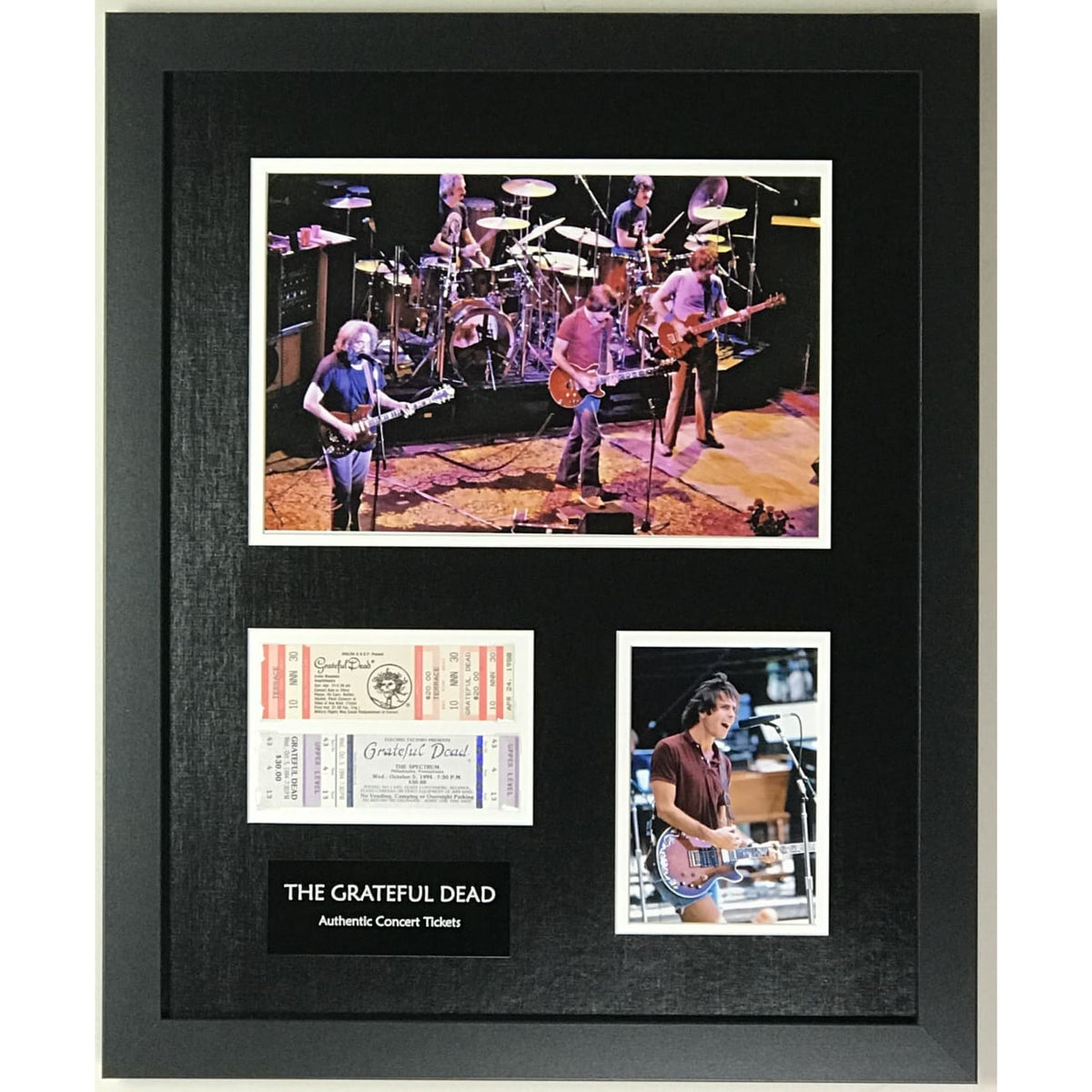The image depicts a framed collage featuring memorabilia from a Grateful Dead concert. The entire piece is enclosed in a black wooden border. The collage contains three main elements: a horizontal photograph at the top showcasing the full band with five musicians on stage, where three members are in the front row with guitars, and two drummers can be seen in the background. Below this, on the left, there is a white box containing two concert tickets, the top ticket adorned with red stripes and the bottom with blue stripes. To the right of the tickets, there is a close-up photograph of a guitarist and vocalist dressed in a brown shirt, holding his guitar and singing into a microphone. At the bottom of the collage, a black plaque with white text reads "The Grateful Dead Authentic Concert Tickets."